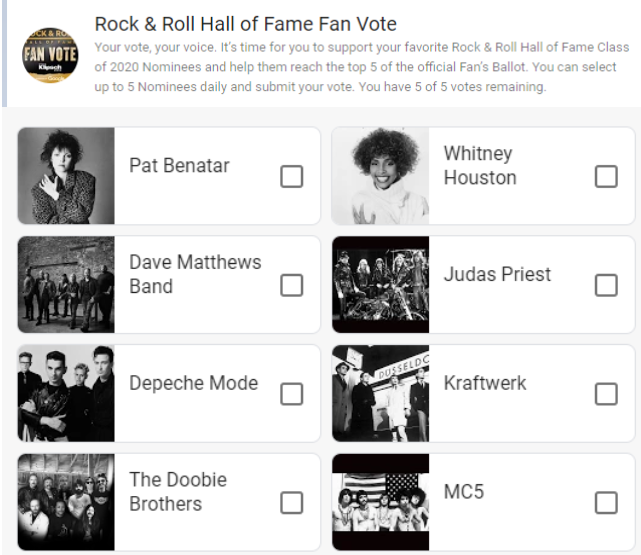At the top of the image, a bold heading reads "Rock and Roll Hall of Fame Fan Vote." Below this, a grey block of text states, "Your Vote, Your Voice. It's time for you to support your favorite Rock and Roll Hall of Fame class of 2020 nominees and help them reach the top five of the official fans ballot. You can select up to five nominees daily and submit your vote. You have five of the five votes remaining."

On the right side of the image, there's a circular emblem with gold text on a black background that reads "Rock and Roll Hall of Fame Fan Vote."

Below this section, the image displays multiple voting options. There are four initial options with names and pictures. On the upper left is Pat Benatar, and to the right of her is Whitney Houston. For both of these artists, the names and faces are clearly visible. Next in line, the image shows the Dave Matthews Band and Judas Priest, where the full bands are depicted.

Additional options include Depeche Mode and Kraftwerk, with images showing the entire bands. The final entries are the Doobie Brothers and MC5, again with images of all the band members. Each voting option features a small empty square for voters to check off their selections.